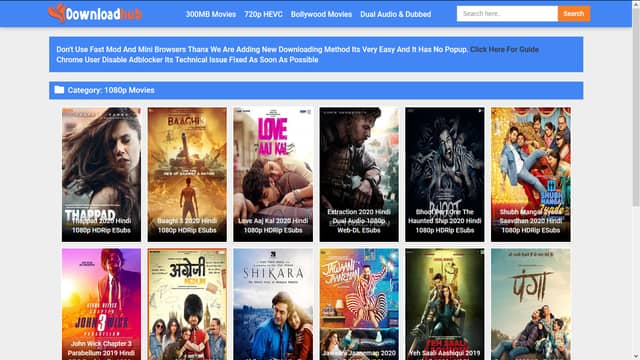The image depicts the homepage of the Download Hub website. At the top left corner, the website's name "Download Hub" is prominently displayed. The word “Download” is in white, while “Hub” is in an orange-reddish color. This is set against a blue navigation bar that spans horizontally across the page.

To the right of the website name, the navigation bar features several categories in white text: "300MB Movies," "720p HEVC," "Bollywood Movies," "Dual Audio," and "Dubbed." Below these categories, there is a search bar with placeholder text prompting the user to enter their query. Adjacent to the search bar, there is a scrolling notification with the message: "Don't use fast mod and mini browser."

Further down, the page designates a category titled "1080p Movies," under which a grid layout displays a list of movie thumbnails. The grid is organized into two rows, each containing six movies, making a total of 12 visible movie options. Among these movies, titles such as "John Wick 3" and "Shakira" are notable inclusions.